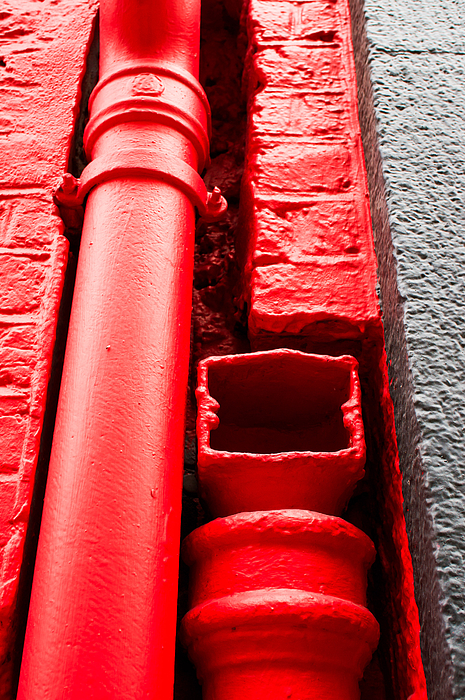This top-down photograph captures a colorful urban scene dominated by a vibrantly edited red pipe system set against a contrasting gray sidewalk section on the right edge of the image. The red pipe, appearing to extend vertically, spans much of the left side of the photo, intertwining with various elements such as a metal brace and open vent-like structure, all painted the same vivid red. Below the pipe, the red-tinted ground seems to have been peeled back, revealing the underlying surface and additional metallic components. The meticulously detailed red-bricked and red-stone surroundings further enhance the attention to the red accents, making the gray sidewalk on the right stand out. The image, with its precise details and striking colors, has a professional quality, evoking the impression that it may have been digitally edited to emphasize the red elements.